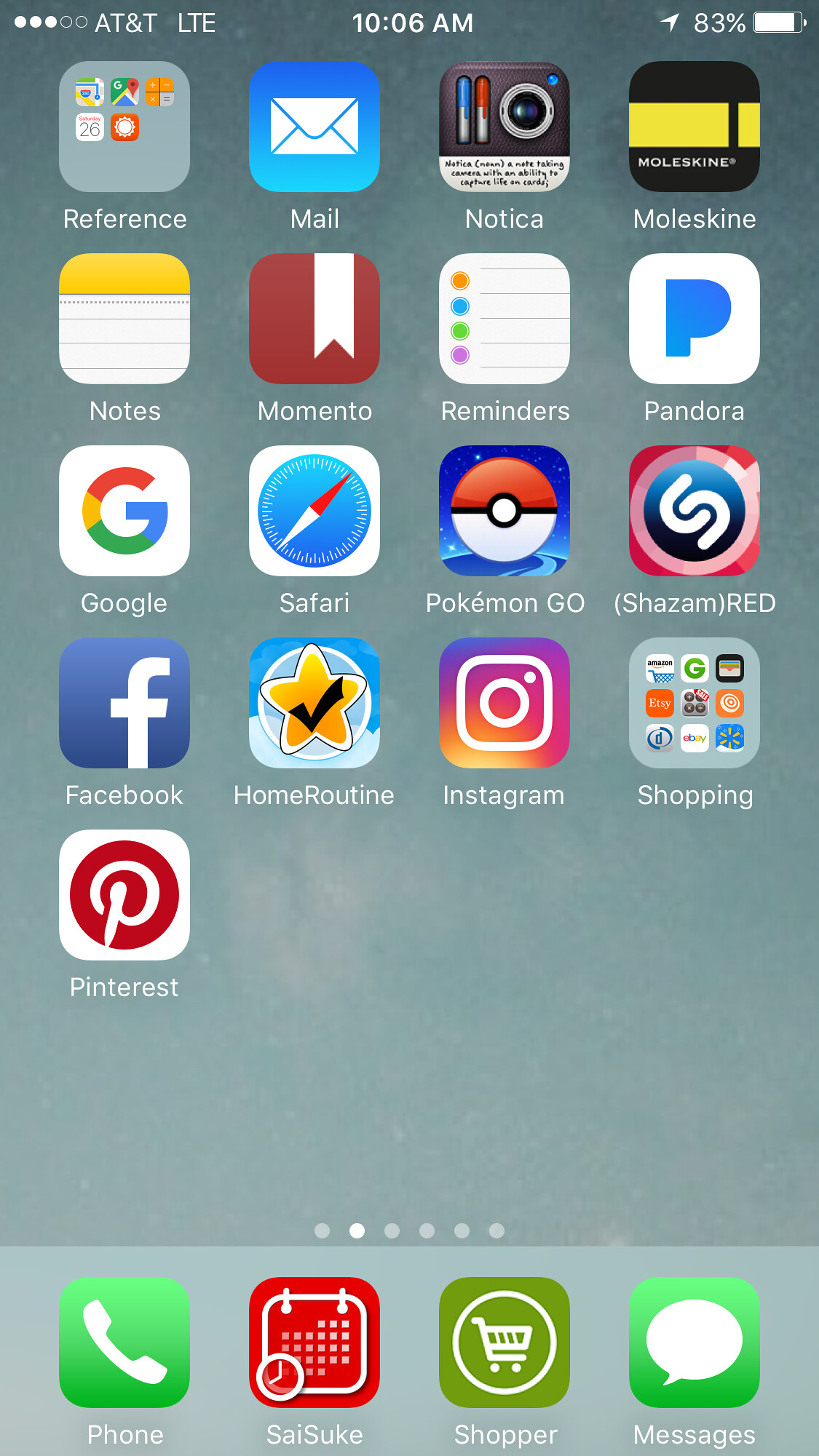Here is a detailed, cleaned-up, and descriptive caption for the given image:

---

This image is a screenshot of a smartphone home screen, displaying various apps. At the top of the screen, the status bar shows "AT&T LTE" as the carrier, the time is 10:06 a.m., and the battery level is at 83%.

The first row of apps contains a folder labeled "Reference," which includes five apps, among which are Google Maps, Clock, and AccuWeather. To the right of this folder, there are three more apps: Mail, Nautica (an app that resembles a camera with markers), and Moleskine (a black app with a yellow bar in the middle and a black bar running through it).

In the second row, the screen displays:
1. Notes (depicted as a white lined paper with a yellow header)
2. Momento (a red or burgundy app with a white ribbon)
3. Reminders (with four colored dots - orange, green, blue, and purple - on the left and lines on the right)
4. Pandora (a large blue "P" on a white background)

The third row features:
1. Google (identified by the multicolored "G" on a white background)
2. Safari (a blue compass with a half-white, half-red dial)
3. Pokémon GO (showing a blue background with a red and white Pokéball)
4. Shazam (with a red background, a blue circle, and a fragmented "S")

The fourth row includes:
1. Facebook (a blue background with a small white "f")
2. Home Routine (a slightly blue background with a clear circle and a yellow star marked with a black checkmark)
3. Instagram (featuring a gradient from yellow to pink with a bit of blue at the top left, a white square, circle, and dot)
4. A folder labeled "Shopping," containing nine apps. Recognizable ones include Temu, Google Shopping (green), and Walmart (blue with a yellow sunburst).

In the fifth row, there is only one app:
- Pinterest (a white square with a pink circle and a white "P")

Finally, at the bottom row (the dock), we have:
1. Phone app (a green background with a white phone icon)
2. SAISUKE (a calendar app with a red background)
3. Shopper (a green background with a white circle containing a white shopping cart)
4. Messages (a green background with a white speech bubble)

---

This caption provides a thorough breakdown of the apps and their respective icons, with clear descriptions for visual identification.